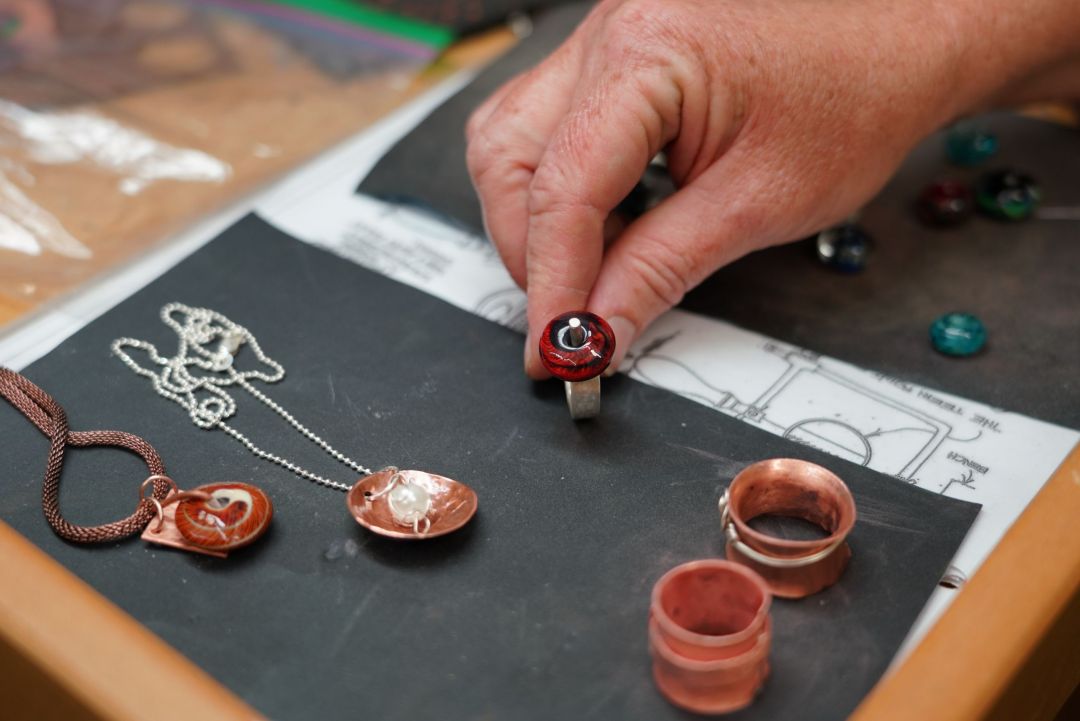In this photograph, a jeweler is meticulously working at a wooden workbench. His hand, emerging from the upper right corner of the image, holds an open silver ring with a red and black stone in place, though the central jewel is currently missing, revealing the ring's prong setting. The ring is positioned above a black mat. The workspace is dotted with various tools and scattered jewels, hinting at the intricate work being carried out. 

In the foreground, there are two necklaces, one featuring a wooden disk with intricate white painting, and the other adorned with white beads and an inverted gold panning bowl-like pendant. Additionally, a gold ring with a unique red, white, and blue yin-yang design, and another jewelry piece with gold and white elements, are visible. A partially visible blueprint peeks through beneath the jeweler's hand, which rests atop the black mat, contrasting against the dark-colored paper on the table. The background is filled with a mix of brown, white, blue, and green elements, possibly other tools or materials, suggesting an organized but busy craftsman’s workspace. There’s also an impression of a pawn shop environment due to the assortment of items and the setup.